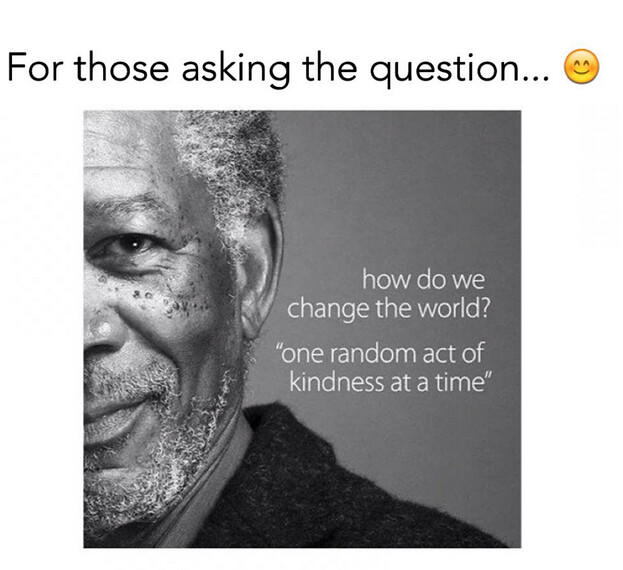The image is a black-and-white photograph featuring a close-up, square-format portrait of the renowned actor Morgan Freeman. The photo captures the right half of his face, from his nose to his ear, and extends from just above his forehead to slightly below his chin, including a part of his shoulder, which is clad in a black collared shirt. Morgan Freeman is depicted with a subtle smile, his familiar features rendered in a detailed grayscale. On the left side of the image, against a clean gray background, there is a prominent, uplifting quote in small, white text: "How do we change the world? One random act of kindness at a time." This inspirational message stands out in its simplicity, effectively paired with Freeman's thoughtful expression to evoke a sense of compassion and positive change.